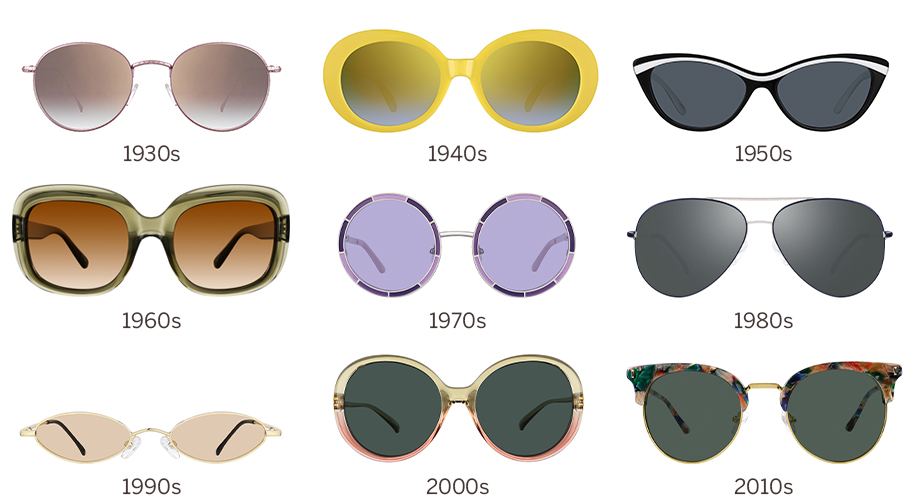This image showcases a meticulous display of nine different pairs of sunglasses, each representing a distinctive style from each decade between the 1930s and the 2010s, arranged in three stacked rows against a plain white background. The top row features the 1930s gray aviator-style glasses, the 1940s with wide-brimmed yellow-rimmed glasses with shaded interiors, and the 1950s black cat-eyed frames with a characteristic white stripe across the top. In the middle row, there are the 1960s wide-rimmed brown sunglasses, the 1970s round, circular glasses with a lavender tint, and the 1980s triangular-shaped sunglasses with a gray tint. The bottom row displays the 1990s narrow golden oval-shaped glasses, the 2000s large plastic-framed glasses with green on the top and pink on the bottom, and the 2010s large frames with a multicolored design featuring green, white, and red along the top of the thick frame. This illustrative array serves as an excellent reference for the evolution of sunglasses over the decades, emphasizing the changes in size and style across the eras.